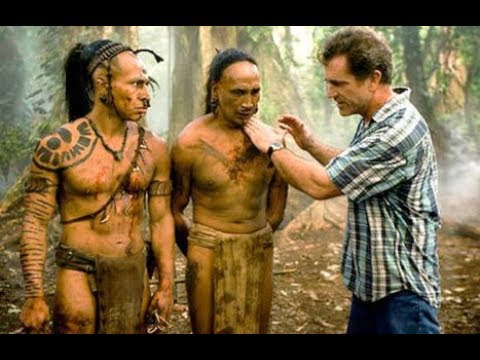In this still frame from the making-of documentary for the film "Apocalypto," directed by Mel Gibson, we see Mel Gibson on the right wearing a short-sleeved plaid shirt and blue jeans, standing in a misty forest. He appears to be giving direction to two Indigenous warriors who stand to his left. Both men have long black hair pulled back into ponytails and are bare-chested, dressed in brown loincloths and smeared with dirt and blood. The man on the right of the warriors, whom Mel is touching on the chest, has a large bird tattoo prominently displayed. The man on the left has intricate tribal tattoos on his shoulder and upper arms. The image captures the immersive and gritty environment of the film set, with a focus on the detailed appearances and costumes of the characters.